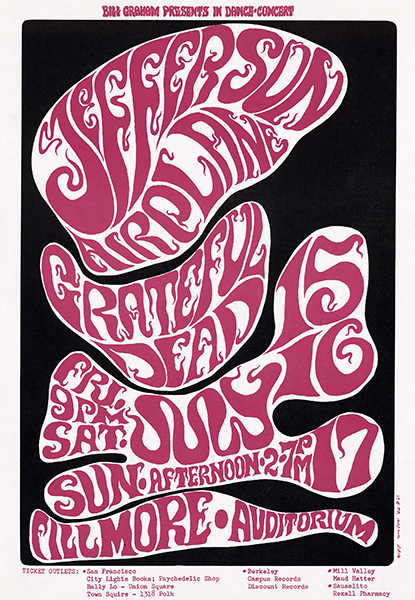This is a highly detailed, psychedelic poster, likely from the 1960s, advertising a series of concerts. The poster features a small vertical rectangle with a black background and ornate, irregular white shapes containing vibrant red and purple text. Prominently displayed within the largest white bubble in a stunning 60s psychedelic font is "Jefferson Airplane," with another curved shape below it announcing "Grateful Dead." Alongside these names, the number "15" is visible, indicating the dates and times of the performances: Friday at 9 PM, Saturday, July 16th, and Sunday afternoon, July 17th at 2-7 PM. These concerts are scheduled to take place at the Fillmore Auditorium, as stated in a bold section at the bottom of the poster. Notably, the bottom half of the poster lists ticket outlets in typed font, mentioning locations like San Francisco, Berkeley, Mill Valley, and Sausalito. The topmost section of the poster, adorned with another psychedelic font in purple, reads "Bill Graham Presents in Dance Concert," framing the entire advertisement with a nostalgic 60s flair.